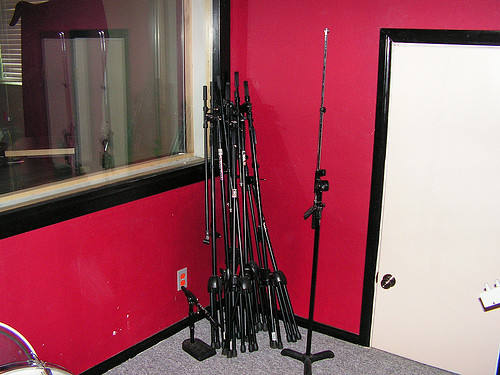This color image captures the inside of a business office or possibly a recording studio, featuring a room with striking red walls and black trim. The scene is centered on the back corner of the room. On the left side, there is a large, transparent window with a white frame and black border, showing a view into another room that has additional windows and possibly some Venetian blinds. Below and beside this window, leaning against the red walls in the corner, are numerous black mic stands, reminiscent of equipment stands that could be used in a studio setting.

On the right side of the room, there's a white door with the handle placed unusually low, about a foot or knee level from the floor, suggesting it might be designed for a very short person or possibly has a unique function. This door also features black trim. The floor of the room is covered with a gray low-pile commercial carpet. Notably, one of the microphone stands is fully extended with legs splayed out, implying it is ready for use. The overall detailed view, from the red walls to the door and the mic stands, offers a glimpse into a professional space equipped for audio or visual recordings.